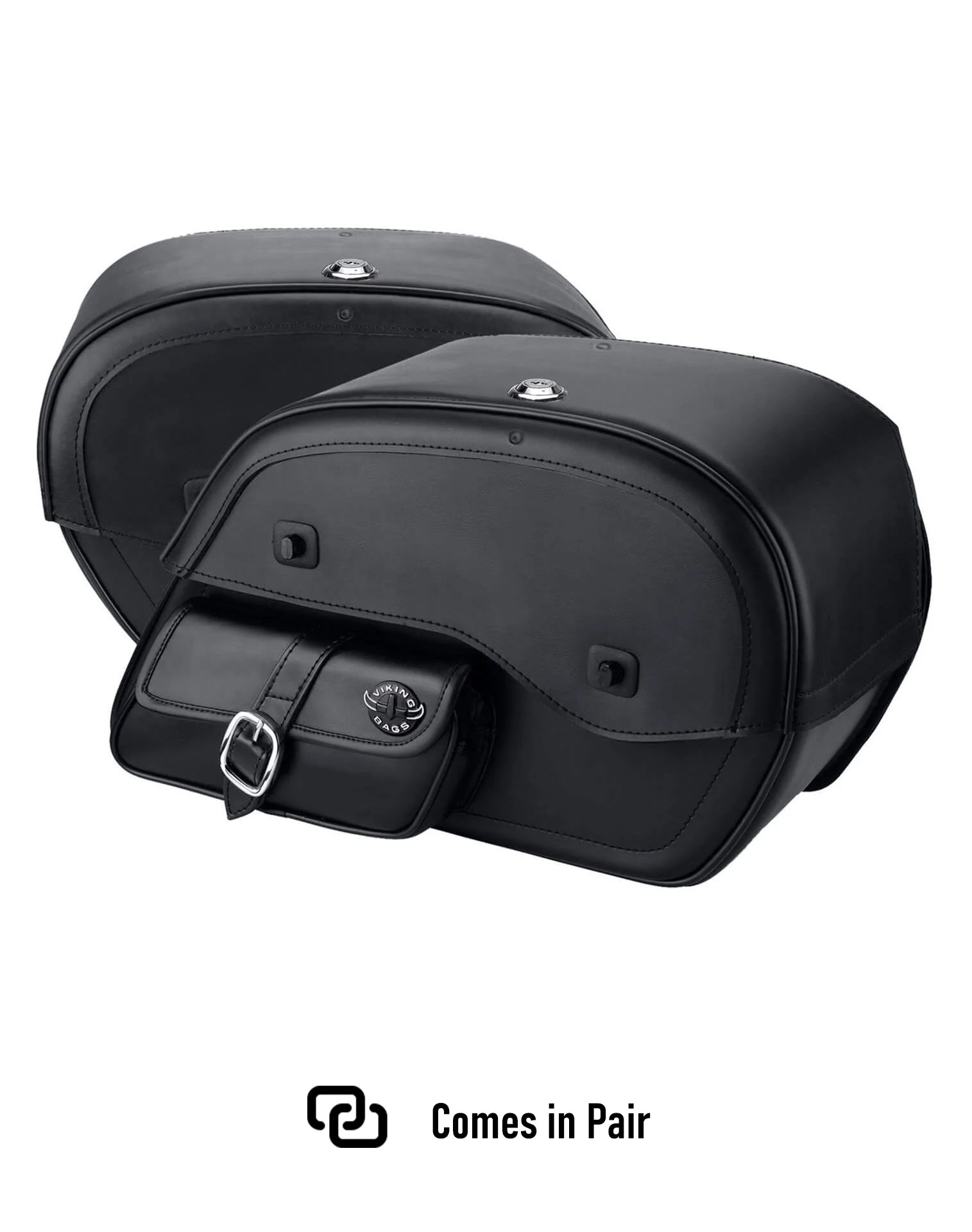The image features a pair of black leather bags with a hard-shelled, oblong design. These bags, potentially side or saddle bags for a motorcycle, are displayed against a completely white background. Each bag has a flap that closes with a silver lock at the top. Below the main body, they house smaller pockets—one of which has a leather strap and a metal clasp. On one bag, there's branding that reads "Viking Bags" in white letters. At the bottom of the image, there’s a logo of interlocked chain links next to the words "comes in pair" written in black. The bags appear identical, suggesting they are designed to be used as a mirrored pair, possibly on either side of a motorcycle.